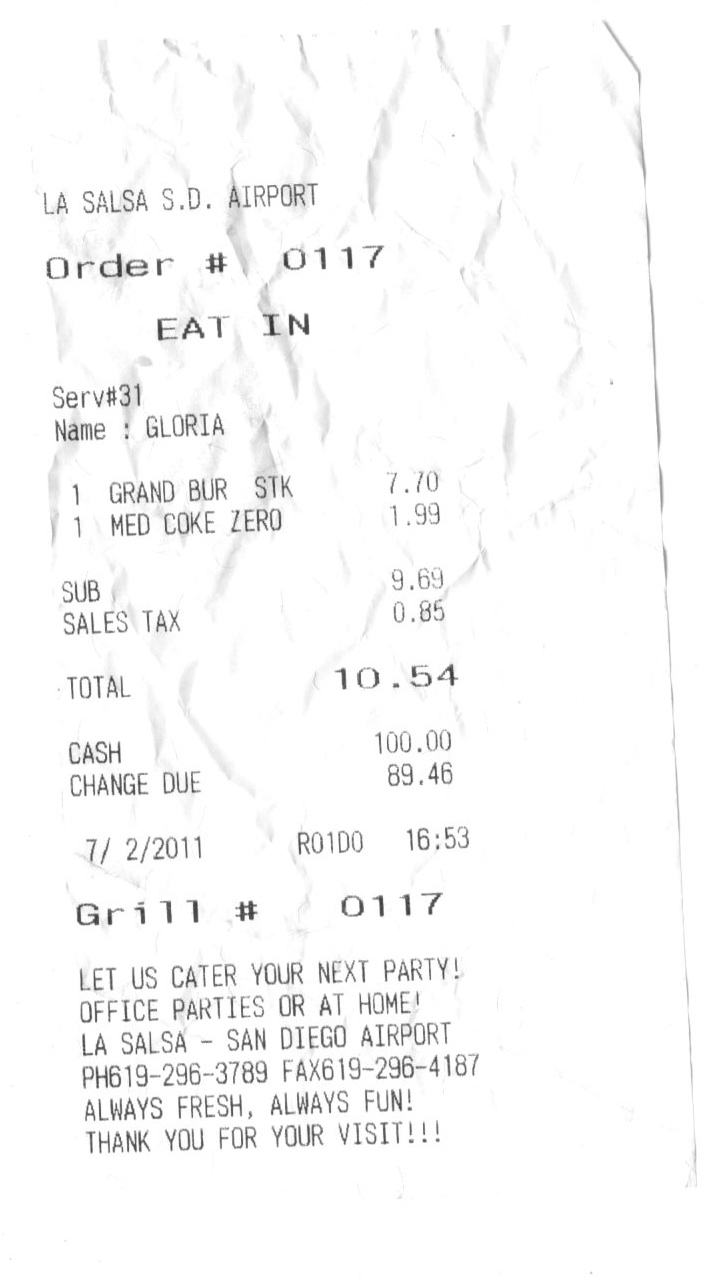A white receipt is placed on a white paper background from a location called "La Salsa SD Airport." The order number is 0117 and the server is identified as Gloria, who appears to be serving at grill number 0117. The items ordered include a Grilled Burrito Stick priced at $7.70 and a medium Coke Zero for $1.99. The subtotal for these items is $9.69, with a sales tax of $0.85, bringing the total to $10.54. The payment was made with a $100 bill, resulting in a change of $89.46. The transaction took place on July 2, 2011, at 4:53 PM.